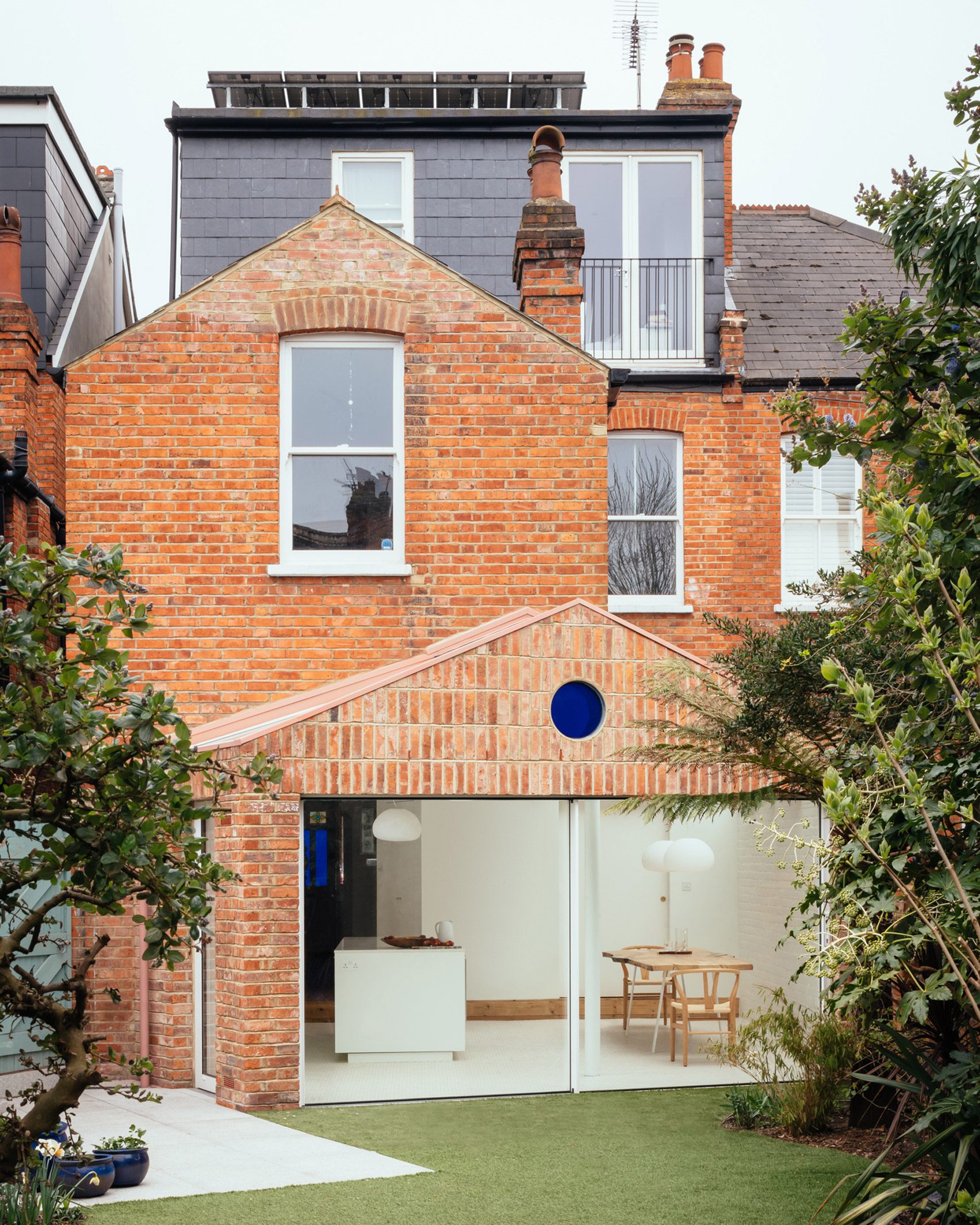This photograph, taken on a cloudy daytime, showcases a large multi-story red brick house centrally positioned within the frame. The scenic outdoor setting features green grass in the foreground and trees flanking both sides of the house. The bottom level of the house includes expansive floor-to-ceiling sliding glass doors that reveal a bright kitchen area with white walls and a white floor. Inside, a brown kitchen table with two chairs is visible under a large hanging light, alongside a kitchen island with another light fixture above it. A distinct blue dot marks the brick exterior near this section. Moving up, the house has a second story with three white-trimmed windows. The topmost floor, integrated into the roof, features small windows on the left and a petite balcony. The roof itself is adorned with gray shingles, solar panels, and at least two chimneys, as well as an antenna.